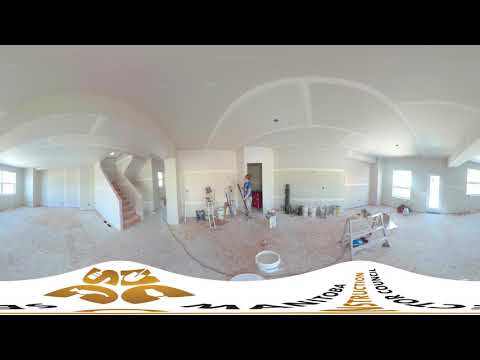The image depicts the interior of a large, white living space under construction or being decorated, characterized by its elegant barrel vault ceilings and bright natural light pouring in from open windows. Central to the scene is a woman, possibly a cleaning lady or worker, standing near an open doorway, holding what appears to be a broom, mop, or paintbrush. Surrounding her are various items including a stepladder, several white buckets or tins, likely containing paint or plaster, and scattered around the white, slightly sloped floor which has a subtle pink hue in some areas. A staircase, also white with pink-tinged steps, leads up to the second floor. At the bottom of the image, a banner with partially legible gold and black writing possibly reads "Manitoba Construction Council," suggesting it could be an image from a construction or work group project.